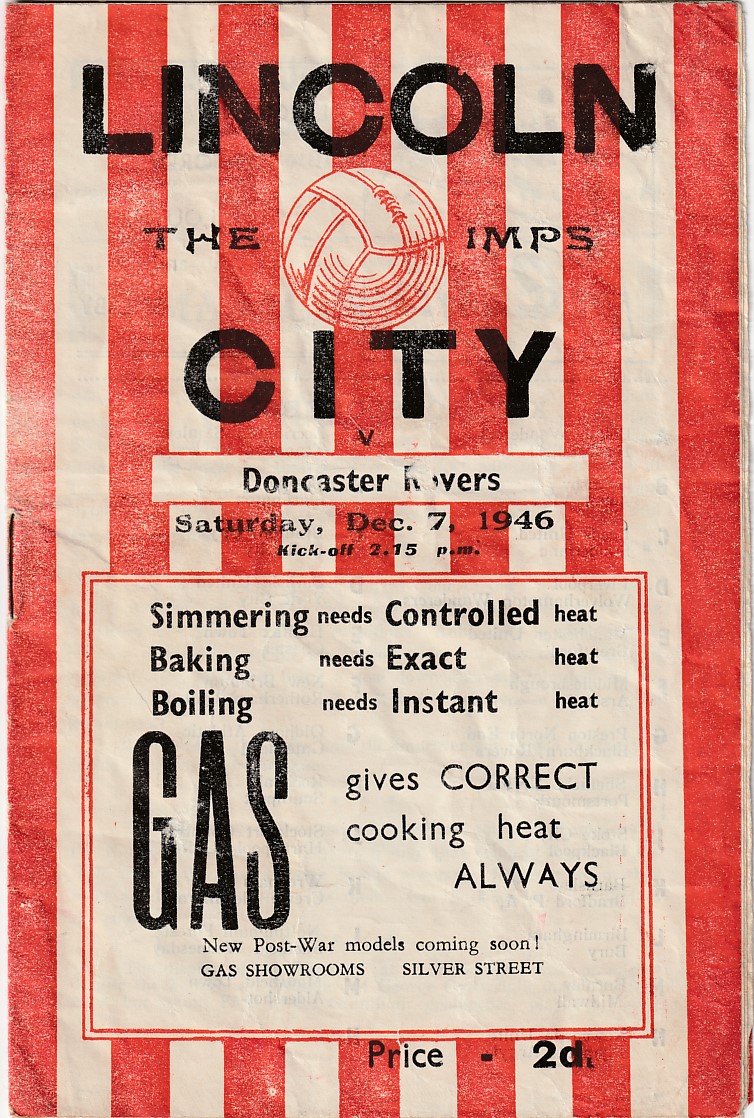This is the cover of a vintage game day program from an English football club match between Lincoln City and Doncaster Rovers, dated Saturday, December 7th, 1946, with kickoff at 2.15 p.m. The background features vertically striped red and white aged paper, giving it a worn and wrinkly appearance. At the top, in bold black text, it reads "Lincoln," and below this, the text "The I.M.P.S. City" is arranged around an illustration of a soccer ball, representing Lincoln City's nickname, "The Imps." Further down is a white rectangle with "Doncaster Rovers" printed inside it. An advertisement occupies the bottom half of the cover, with a white square bordered in red and black text that states: "Simmering needs controlled heat. Baking needs exact heat. Boiling needs instant heat. Gas gives correct cooking heat always. New post-war models coming soon. Gas showrooms, Silver Street." The program price is listed at 2d, indicating its historical context.